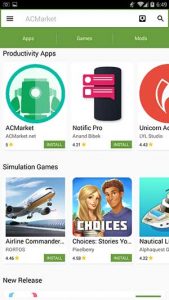The image depicts a screenshot from the AC Market app store, showcasing various downloadable apps and games. At the top, there's a status bar displaying the current time and several icons, which are somewhat blurry but include a nearly full battery indicator and internet connectivity status. Below this, on a white background, the title "AC Market" is prominent. Flanking this title are clickable icons: a magnifying glass for search on the right and a hamburger menu (three horizontal bars) on the left.

Beneath the title, on a green background, the word "Apps" is visible, though the text on either side is too blurred to be legible. Below this, the category "Productivity Apps" is highlighted, featuring apps like AC Market itself, Notific Pro, and an app whose name starts with "Unicorn" but is cut off from the picture. Each of these apps has a green box next to it, indicating that they can be installed. Notific Pro has a rating of 4.31, and the Unicorn app has a rating of 4.42, both marked with yellow stars.

Further down, under the category "Simulation Games," the image displays titles such as Airline Commander—depicting a plane taking off—with a rating of 4.46, and Choices: Stories You Play—showing a male and female character side by side—with a rating of 4.58. Additionally, there's a glimpse of a nautical-themed game involving a boat, somewhat cut off, with a rating of 4.22. The games' ratings are also accompanied by yellow stars.

Finally, the bottom left corner features a label that reads "New Releases," marking a section likely dedicated to the latest available content.